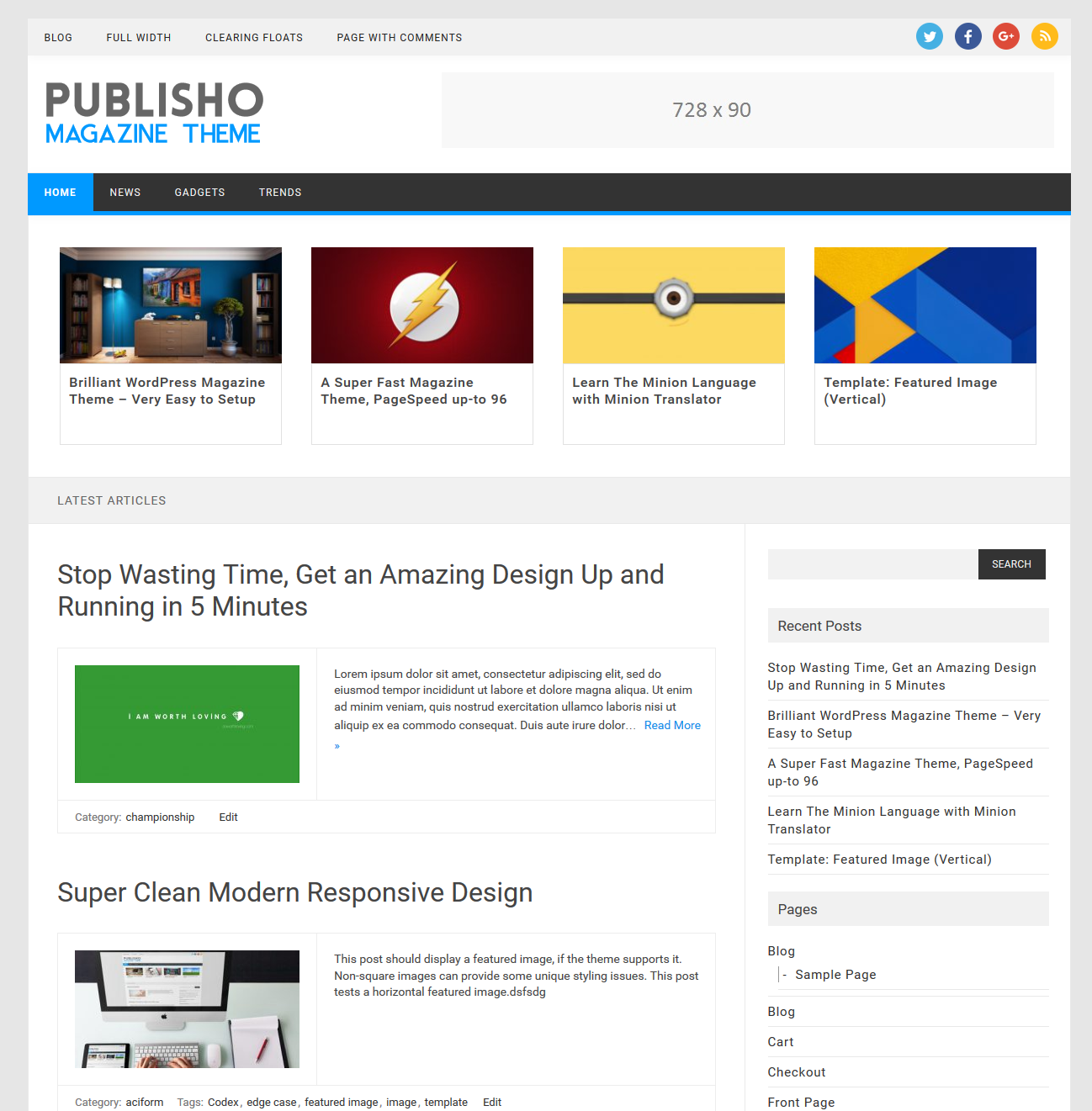**Publish Show Magazine Theme Homepage**

At the top of the page, the title "Publish Show" is boldly written in black, followed by "Magazine Theme" in blue letters. Just beneath the header, a navigation bar offers links to Home, News, Gadgets, and Trends, with Home currently selected.

The main section of the page features four prominently displayed pictures, each associated with key themes:

1. **Brilliant WordPress Magazine Theme**: A visually appealing image accompanied by the tagline "Very easy to set up."
2. **Super Fast Magazine Theme**: An image stating "Page speed up to 96."
3. **Learn the Minion Language with Minion Translator**: A picture linking to information about the Minion Translator.
4. **Template, Featured, Image, Vertical**: This block showcases a vertical image template.

Beneath these featured sections, there is a headline "Latest Articles," introducing two articles:

1. **Stop Wasting Time, Get an Amazing Design Up and Running in Five Minutes**: This article is accompanied by an image with the text "I am worth loving" in white letters against a green background.
2. **Super Clean, Modern, Responsive Design**: The article discusses the importance of non-square images and features a horizontal image of a person typing on a computer, with a notepad and a cell phone beside them. The caption mentions that this post should display a featured image, as supported by the theme.

On the right-hand side of the page, additional features include a search bar and a section titled "Recent Posts," highlighting other articles. There are options for navigating to different pages, including Blog, Sample Page, Cart, Checkout, and a link to the Front Page.